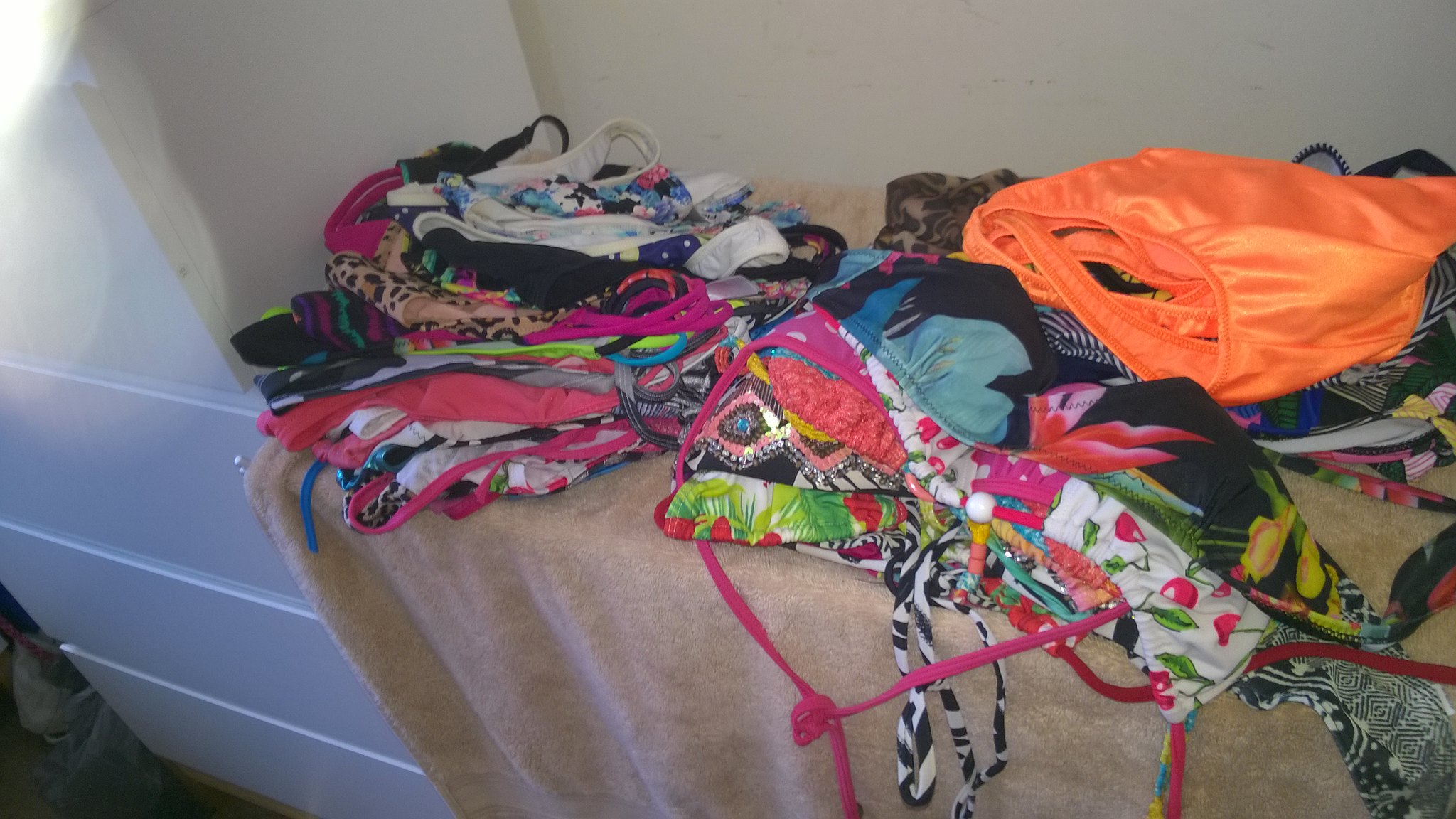This color photograph portrays a white dresser with multiple drawers. The top surface of the dresser is crowded with a light velvet pinkish blanket or large towel, upon which piles of women's bathing suits are stacked. The diverse collection features a variety of styles and prints, including solid colors and vibrant patterns. Notable items include a shiny orange swimsuit on the top of one pile, black swimsuits adorned with blue hibiscus-shaped flowers and bird-of-paradise prints, a white bikini with a cherry pattern, and black and white zebra-striped designs. Some swimsuits feature geometric patterns and vibrant zigzag stripes in electric green, hot pink, and blue. The swimsuits are not new; they appear to have been worn and washed, suggesting the setting might be a laundry room. A light flare in the upper left corner partially obscures the image. The bottom left corner shows a bit of beige carpet, reinforcing the domestic context. There are at least three notably tall stacks of suits, though it’s difficult to determine the exact number.